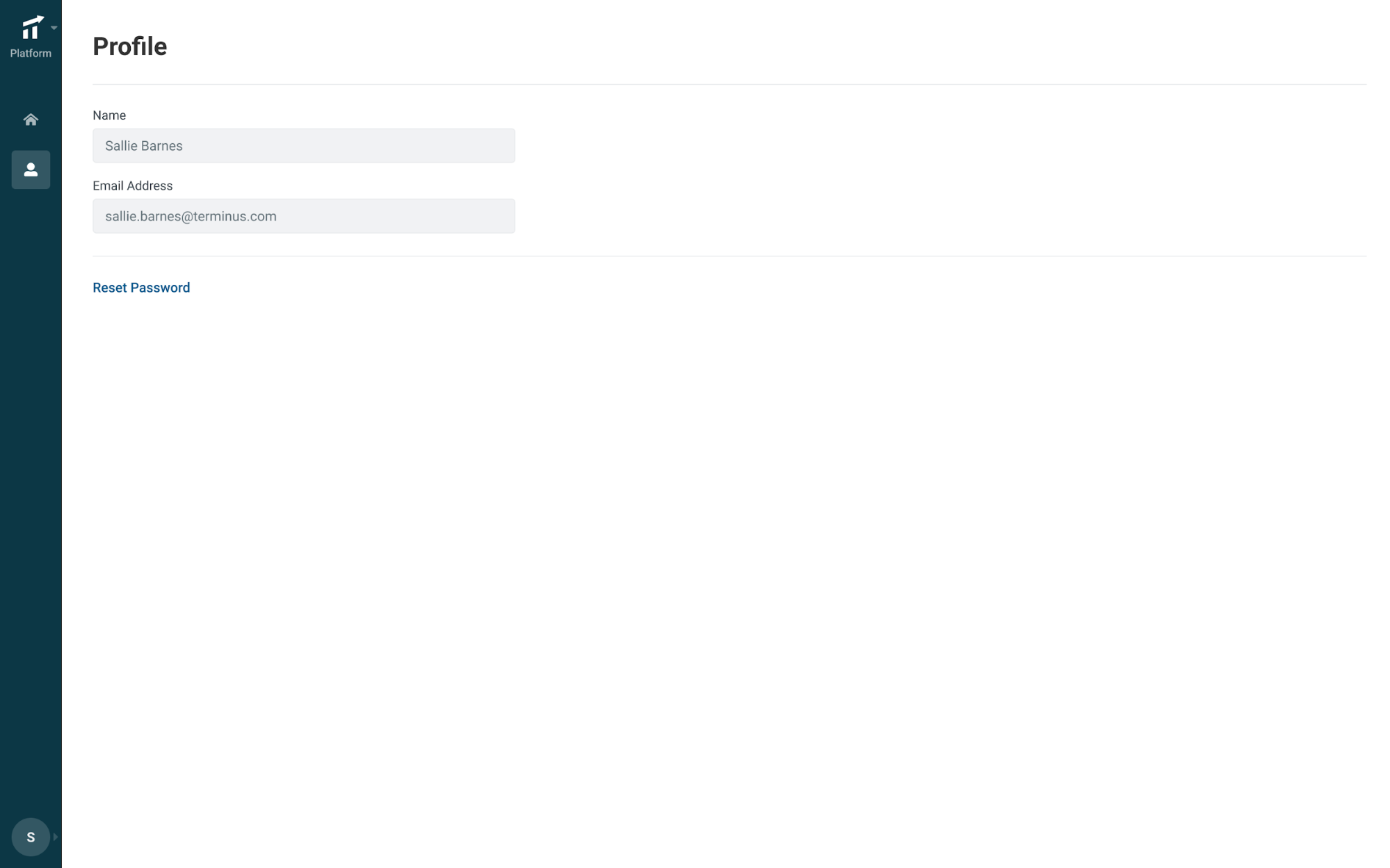The image depicts a webpage that appears to be under construction, characterized by its minimalistic design. The interface features a prominently displayed logo in the top left corner, consisting of an arrow pointing diagonally upwards, supported by small foundational elements. Below this logo, on a dark blue navigation bar along the left side of the screen, are two buttons labeled "Home" and "Profile." 

Upon clicking the "Profile" button, the page reveals fields for a user’s name and email address, which contain placeholder text—specifically, the email address "sally.barnes.com." There is also a "Reset Password" button directly below these fields. The remainder of the page is dominated by white space, indicating its incompleteness. 

At the bottom of the dark blue navigation bar, there is a letter "S," presumably representing the user's initial, which would likely change according to the user's first name. The generic and placeholder nature of some elements, such as the platform's name and the user details, suggests that this webpage is still in its developmental stages.